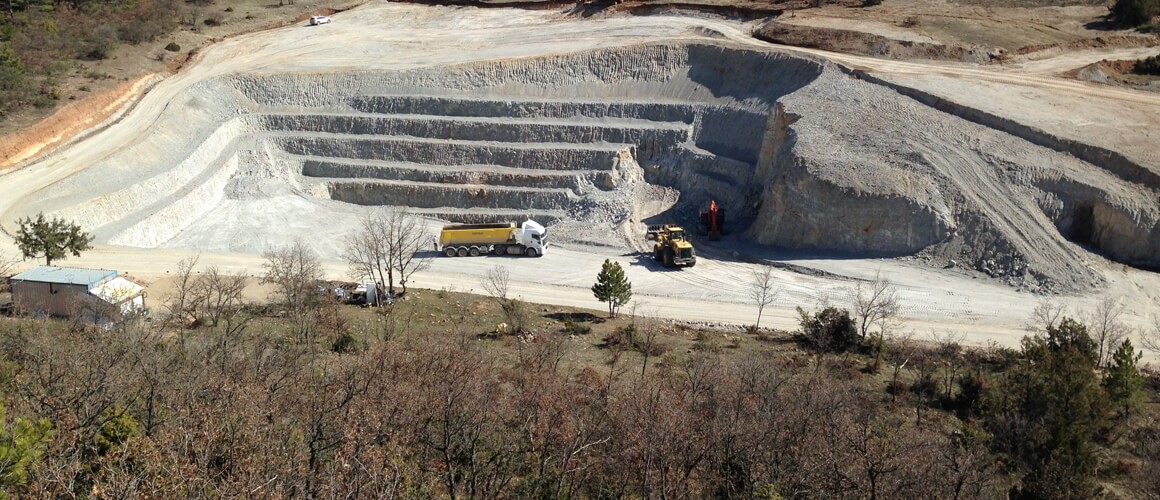The image captures a panoramic view from atop a hill, overlooking a light gray gravel pit at a construction site. The foreground is filled with trees, some bare, others with brown leaves, and a few retaining green leaves on the lower right. Centrally located, the gravel pit features large, step-like terraces etched into its sides for material excavation. At the bottom, a prominent yellow and white dump truck stands alongside an orange track hoe, hinting at ongoing construction work. The rock wall’s upper edge is elevated, bordered by verdant green and brown areas, possibly dirt and additional trees. Bright daylight, despite the absence of the sky in the photograph, illuminates the entire scene, indicating the presence of the sun. A camper is also visible near the trees and grassy slopes on the hill opposite the pit.